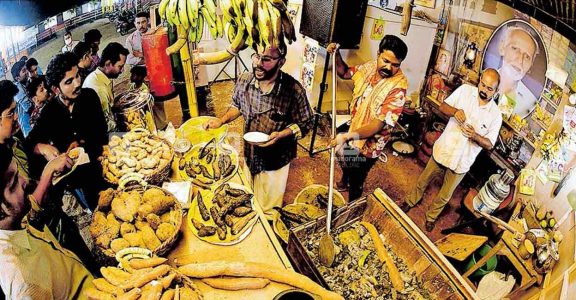This photograph vividly captures a bustling marketplace, likely situated in India or Malaysia, characterized by its vibrant and lively atmosphere. Central to the scene is a vendor in a plaid shirt and glasses, positioned behind a table laden with a variety of food items. He is actively engaged in serving food to a number of customers, predominantly Indian men, who are lined up on the left side. Many of these customers hold plates in anticipation. The table is covered with large pans containing assorted foods, ranging from possible meats and vegetables to items resembling potatoes, all tinged in light brown and yellow hues, contributing to the image's overall yellow-toned, almost sepia appearance. 

In the background, another man, donning an orange shirt, is stirring food with a long wooden paddle in what appears to be a large vat. Further behind him stands a man in a white shirt, deeply engrossed with something in his hands. Surrounding this central activity, the environment is packed with food products, and prominently, there are bunches of bananas hanging from the ceiling. The photograph, while detailed and sharp, exudes an immersive quality, portraying a snapshot of daily life in a vibrant marketplace with its rich array of sights and interactions.